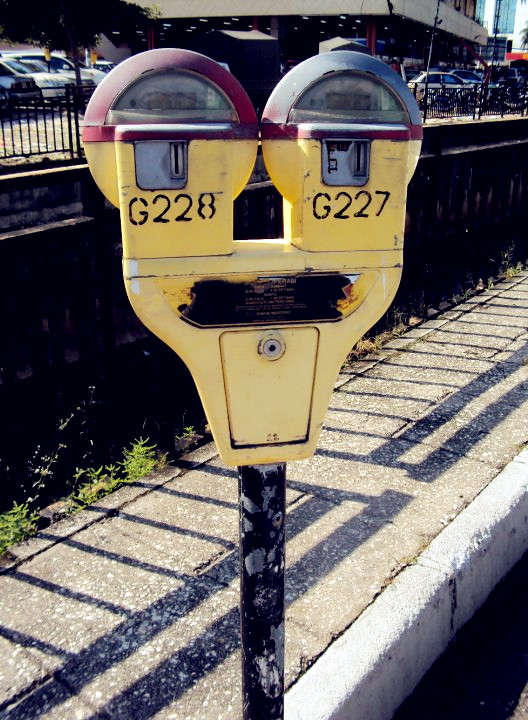This is a vertically oriented outdoor color photograph taken in bright sunlight, capturing an older-style parking meter situated in an urban environment. The parking meter stands prominently in the center of the image, mounted on a black post that shows signs of chipped paint. The meter itself is divided into two sections, one labeled "G228" and the other "G227," both with fogged semicircular glass tops. Its metal body is painted yellow but is scraped and worn, adding to the overall vintage aesthetic. 

Positioned on a concrete sidewalk, the parking meter casts a sharp shadow against a metal fence behind it. This wrought iron fence, black in color, acts as a boundary to a retaining wall just visible in the left background. Above the fence, the scene expands to reveal a city street with rows of parked cars and bikes, indicating a bustling urban setting. The composition highlights both the central meter and the layered textures and structures defining the city's landscape.